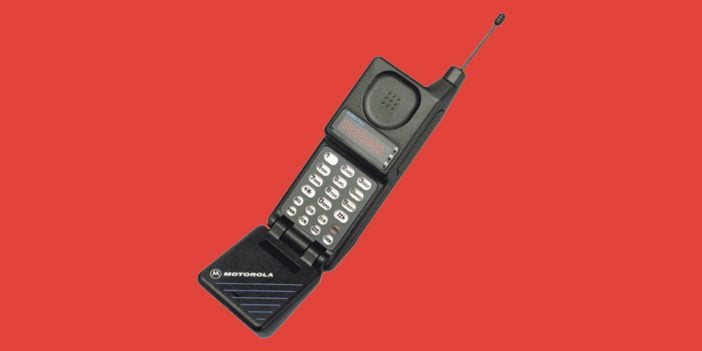Set against a solid red backdrop, the image showcases an old-school Motorola cell phone, likely from the early to mid-1990s. The phone is rectangular and black, featuring a prominent antenna at the top indicative of its age. It includes an LED screen displaying numbers above a keypad with oval-shaped white buttons with black numerals, spanning 1 through 0, as well as the pound key. Below the keypad, there's a part that flips down to reveal the speaker, where you can talk into via a triangular section. The classic Motorola logo, white and encased within a circle, is prominently displayed on the flip part, exuding a nostalgic charm. The phone's earpiece comprises six speaker holes just above the LED screen, completing its retro design.